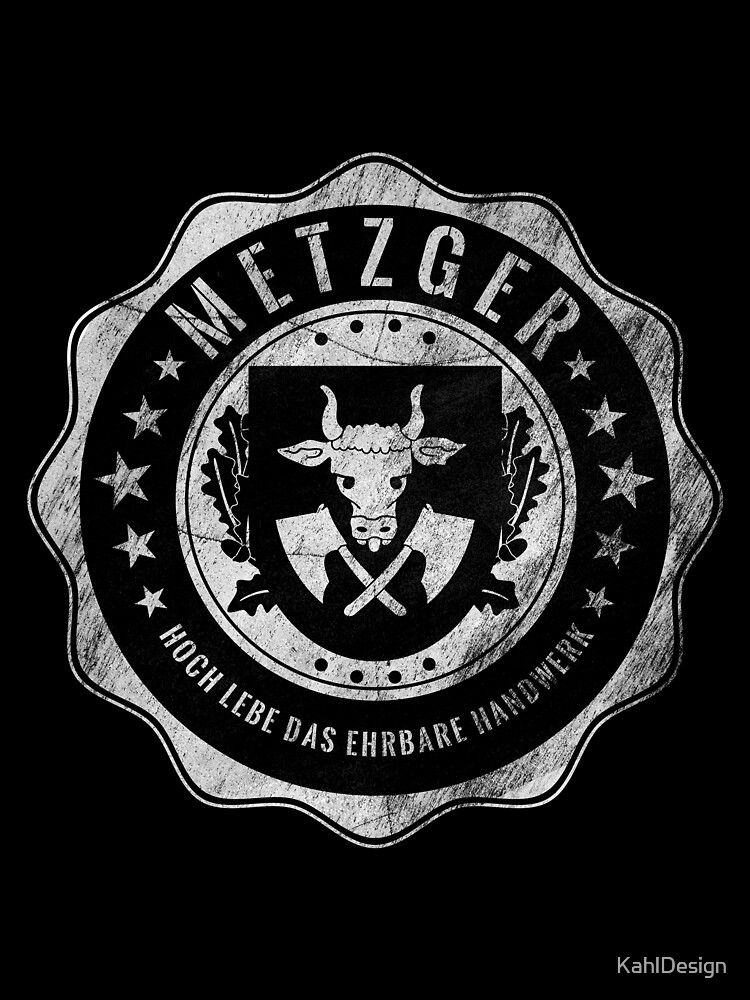The image depicts a vertically oriented rectangular logo set against a solid black background. Dominating the center is a starburst-shaped emblem rendered in white with subtle gray pencil strokes. The centerpiece of the design is a large black circle encircled by numerous small gray stars arranged downward along its perimeter. At the top of this black circle, in off-white brushed letters, is the word "METZGER." Below this, following the curve of the circle, is a phrase in a foreign language that appears to be German, reading "Hock, Lib, Das, Eber." Central to the black circle is a black shield featuring a stylized bull's head, beneath which are two crossed hatchets. Finally, in the lower right-hand corner of the logo, there is a small inscription reading "Kahl Design."